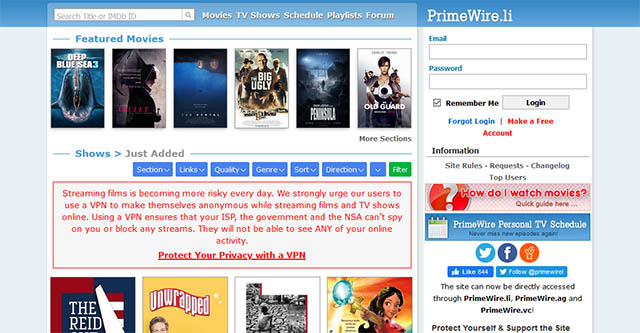This image showcases the layout of the PrimeWire.li website. At the top of the page, there is a search bar prompting users to "search title or IMDB ID," accompanied by a gray magnifying glass icon. Below the search bar, there are navigation tabs labeled "Movies," "TV Shows," "Schedule," "Playlists," and "Forum."

The header also displays the name of the website, PrimeWire.li. Just beneath it, users can find fields to input their email and password, along with a gray login button. There is a "Remember Me" option for convenience, and a link in red text urging users to "Forget Login?" or "Make a Free Account."

In the "Information" section, links are provided for "Site Rules," "Requests," "Change Log," and "Top Users." An advertisement reads, "How do I watch movies? Quick guide here," providing assistance for new visitors.

Featured movies are showcased with various posters, including titles like "Deep Blue Sea 3" and "The Big Ugly." A list highlights recently added shows. Users can refine their browsing with filters for "Selection," "Links," "Quality," "Genre," "Sort," and "Direction."

Social media icons link to the site's profiles on Twitter and Facebook. Additionally, a message informs users that the site is accessible through alternative domains like PrimeWire.ii, PrimeWire.ad, and PrimeWire.vc.

The website's design features gray sidebars and a white background, with a blue header at the top, contributing to its clean and structured layout.